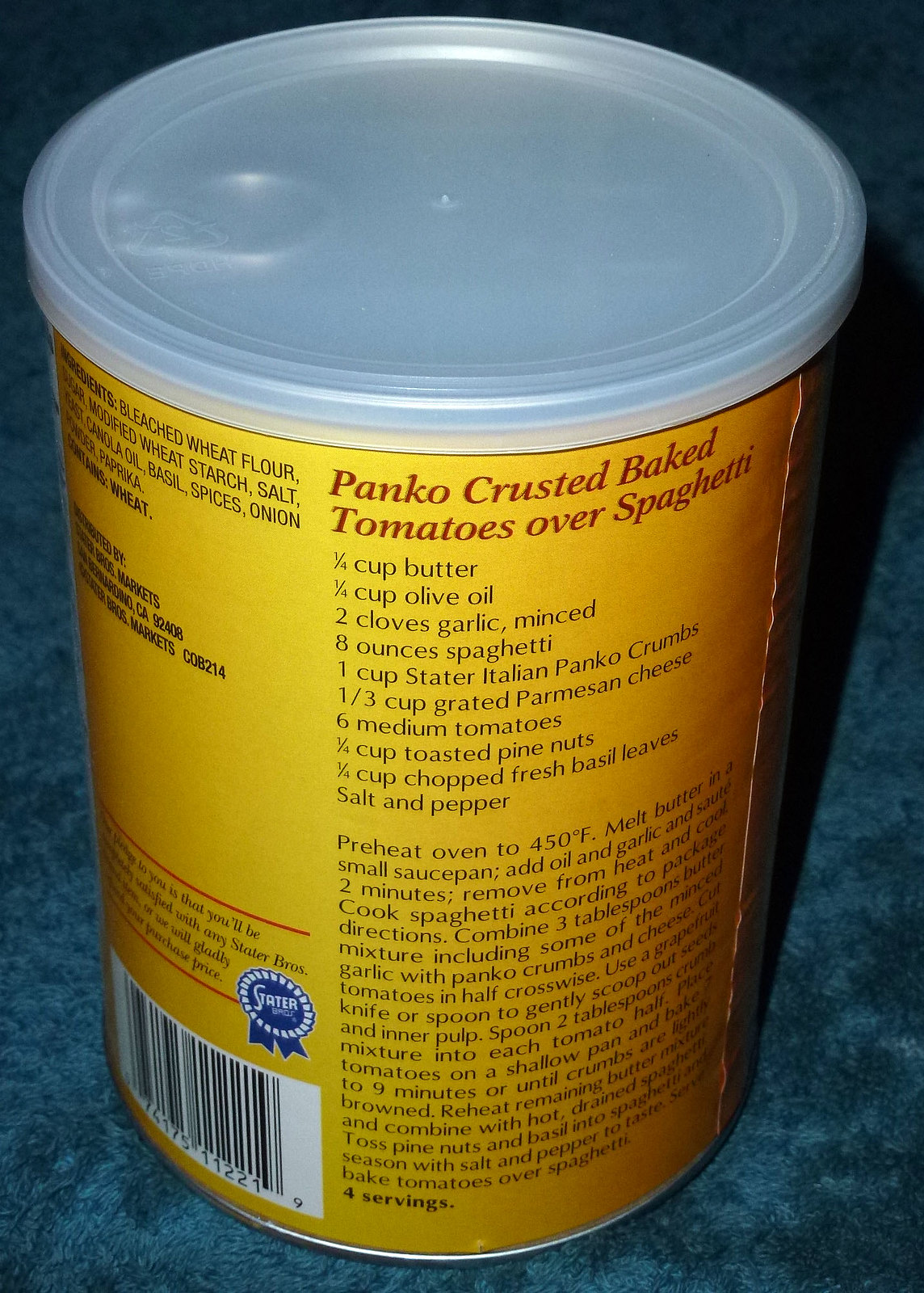This image depicts a product can featuring a semi-translucent plastic top and a metal pull tab lid beneath it. The can's label is a vibrant yellow-orange color, adorned with a recipe title in red letters: "Panko-Crusted Baked Tomatoes Over Spaghetti." Beneath the title, the label provides a detailed recipe with ingredients and instructions, all scripted in black text. On the left side of the label, visible before the can's curvature hides part of it, there is detailed product information and a small blue ribbon seal that reads "Stater" in white letters. The can is placed on a blue carpeted surface, enhancing the visibility of its colors and details.